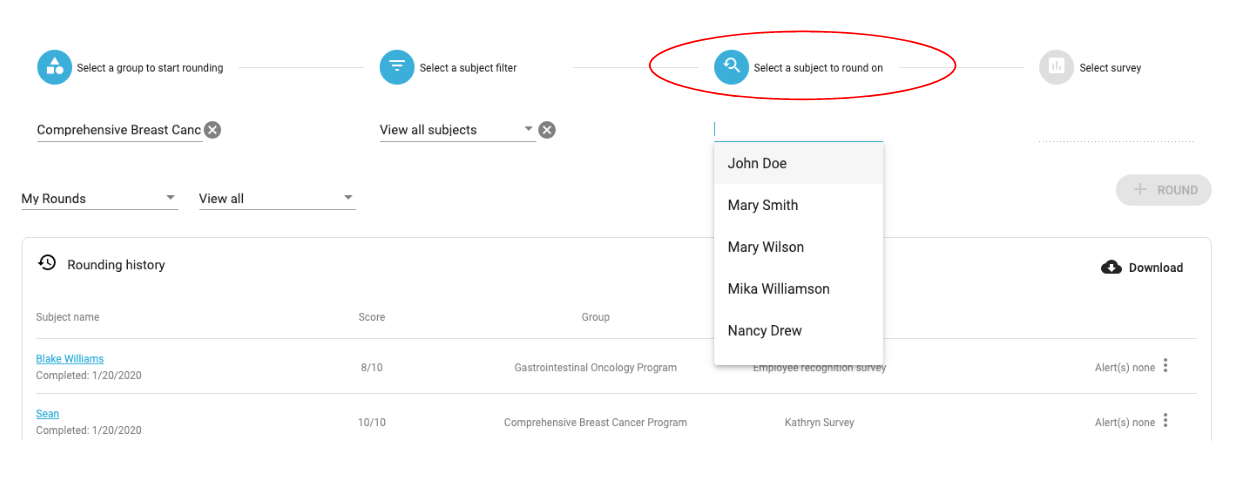**Detailed Screenshot Description:**

The screenshot depicts a user interface designed for managing rounding activities. At the top of the screen, there is a progress bar marked with round blue icons indicating different steps: 

1. **Select a group to start rounding** - Positioned on the left side.
2. **Select a subject filter** - Connected by a line from the first step.
3. **Select a subject to round on** - Connected by a line from the second step.
4. **Select survey** - Connected by a line from the third step.

The "Select a subject to round on" section is highlighted with a red circle for emphasis. Directly below this section, a drop-down menu displays several names: John Doe, Mary Smith, Mary Wilson, Mary Williamson, and Nancy Drew. 

Further down, there is a field labeled "comprehensive breast cancer" with an adjacent X button for easy removal. This is followed by a "view all subjects" drop-down menu, also featuring an X button to the right. Below this, there are two additional drop-down menus labeled "my rounds" and "view all."

At the bottom of the page, the same drop-down menu reappears, again listing the names John Doe, Mary Smith, Mary Wilson, and Nancy Drew.

This detailed layout helps users navigate the rounding process efficiently by offering multiple selection and filtering options.